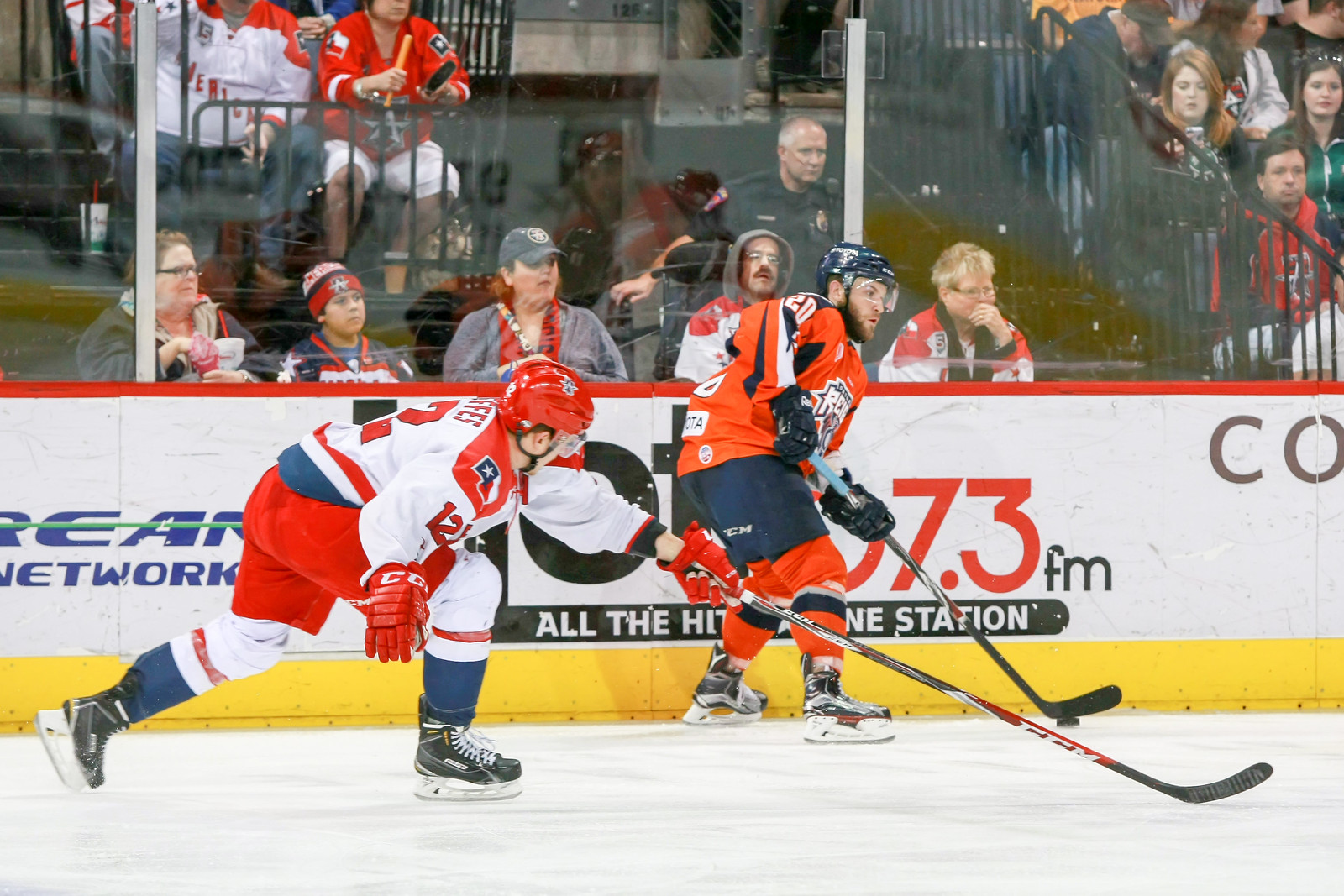In this detailed photograph from a hockey game, we observe two players in the midst of action on the ice. The player on the left, sporting a red and white jersey with blue shorts, has a dark blue helmet and a distinctive reddish beard. He is also wearing black skates and has the puck, poised to make a pass or shoot. The number 20 is emblazoned on his jersey, which features blue stripes and the state of Texas on his shoulder. Positioned next to the barrier, this player is near an advertisement for a radio station with spectators keenly watching the game behind the protective glass.

The second player, wearing a red helmet and an orange, black, and white jersey with number 12, is in red shorts, blue shorts, and orange socks. He has extended his stick towards the puck, seemingly attempting to block the pass or intercept it from his opponent. Both players are captured just off to the side of the goal area, with no sight of the net itself. The background reveals the grandstands filled with fans, some intently watching from behind the glass wall that shields them. The image also highlights a radio station advertisement on the barrier and the yellow rim running along the boards, framing the intense moment in the game.